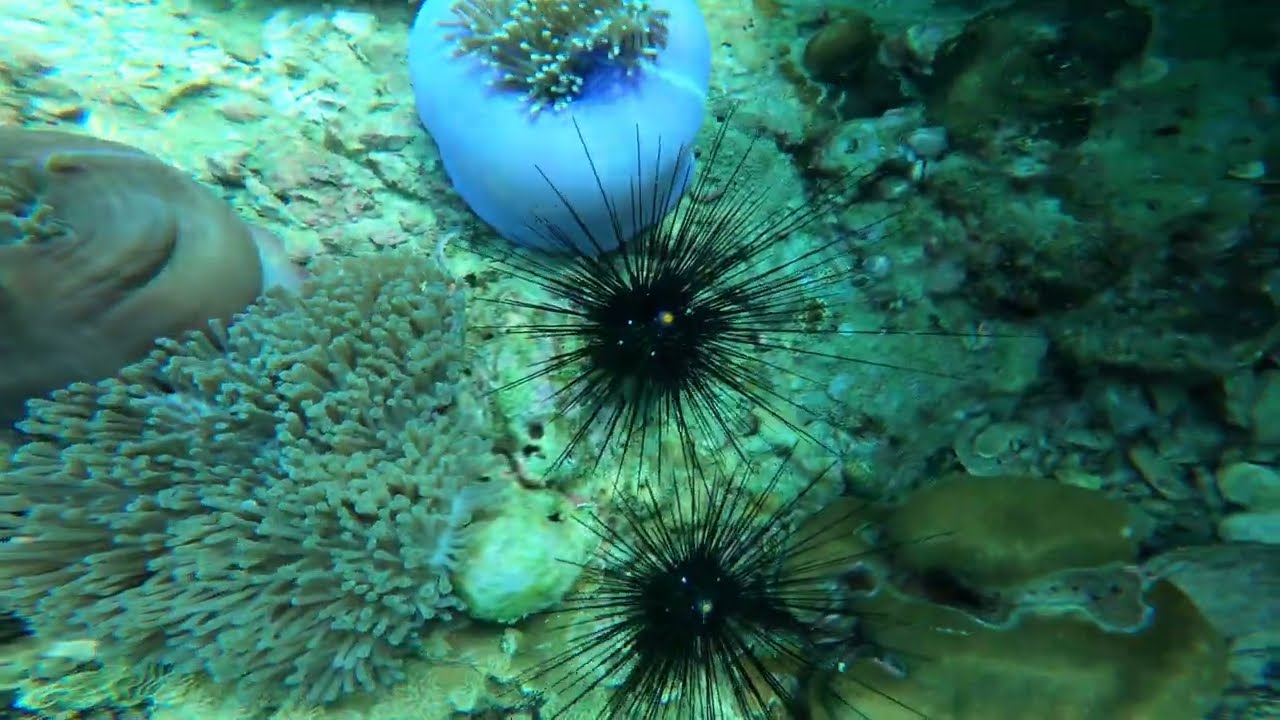This underwater photograph captures the diverse life and vibrant colors of an ocean floor. Central to the image are two black sea urchins adorned with little yellow specks and sharp spines. To their left, a pale green anemone stretches out, resembling a cluster of delicate straws. Above the sea urchins, a striking purplish-blue coral vegetation with additional coral extending upward adds a touch of color. Surrounding the scene is clear, pale-green water that fits into the serene backdrop. Complementing these elements are various underwater structures, such as slimy rocks and spongy-looking formations, including one brown spongy rock. Additionally, there are greenish rocks on the far right side, creating a diverse underwater landscape filled with various textures and life forms. The overall composition highlights the intricate and colorful ecosystem found at the ocean's bottom.